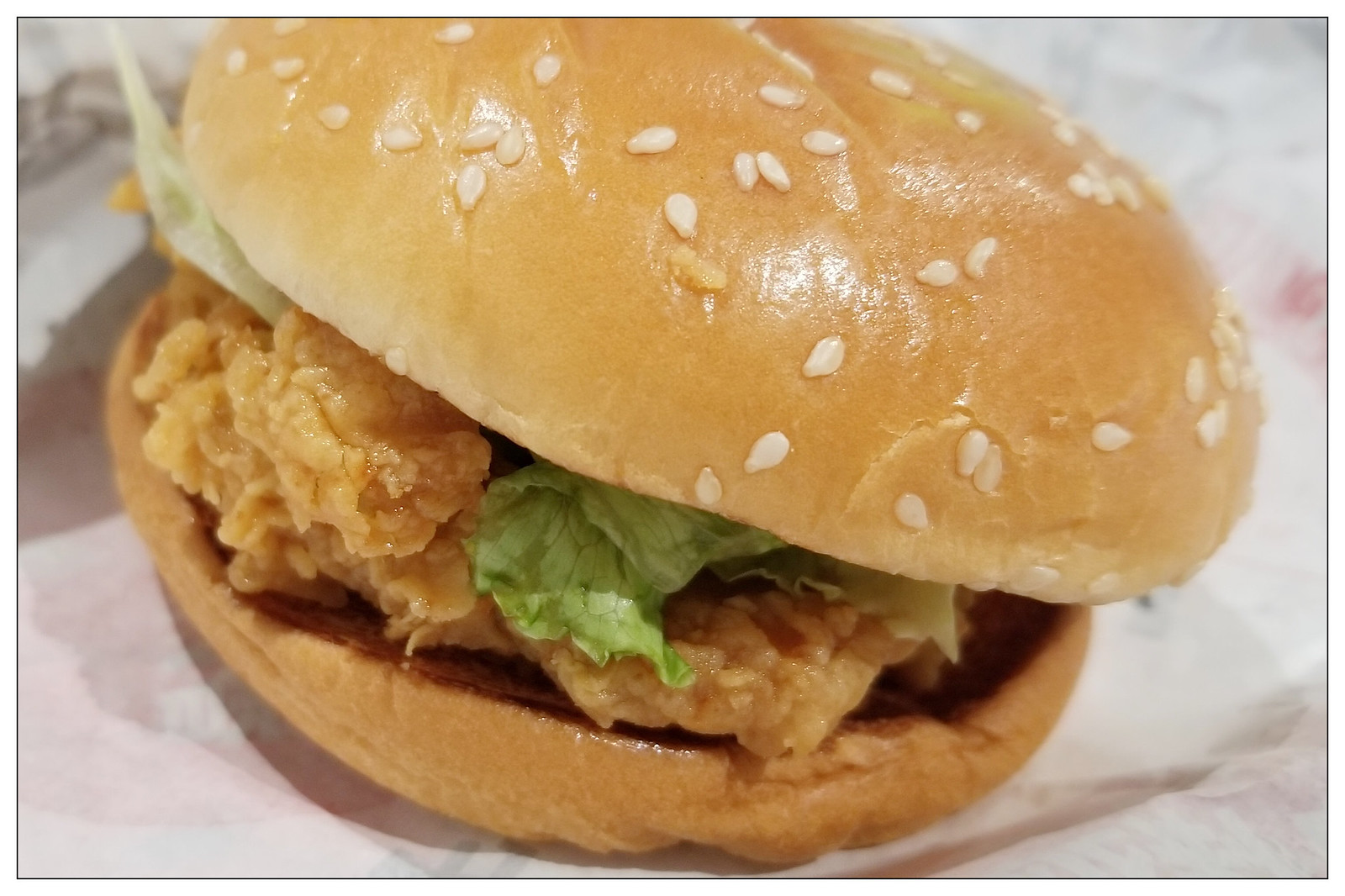The rectangular photograph, approximately four by six inches and bordered with a thin pinstripe of either dark gray or black, features a close-up of a fried chicken sandwich. This sandwich, against a backdrop of white, slightly wrinkled wrapping paper, boasts a golden brown sesame seed bun. The top bun, light golden with white sesame seeds, sits above a layer of crispy fried chicken, potentially fish, with a thick, light brown coating. Peeking out from the sandwich is a wilted piece of green lettuce and a small corner of cheese. The bottom bun appears a bit soggy but toasted. Shadows in the image suggest that the light source is positioned above and behind the sandwich. The glossy appearance of the bun and fried chicken adds a sheen to the overall presentation, making it quite vivid within the photograph. The burger is prominently featured, with the top bun partially cut off but the bottom bun fully visible.